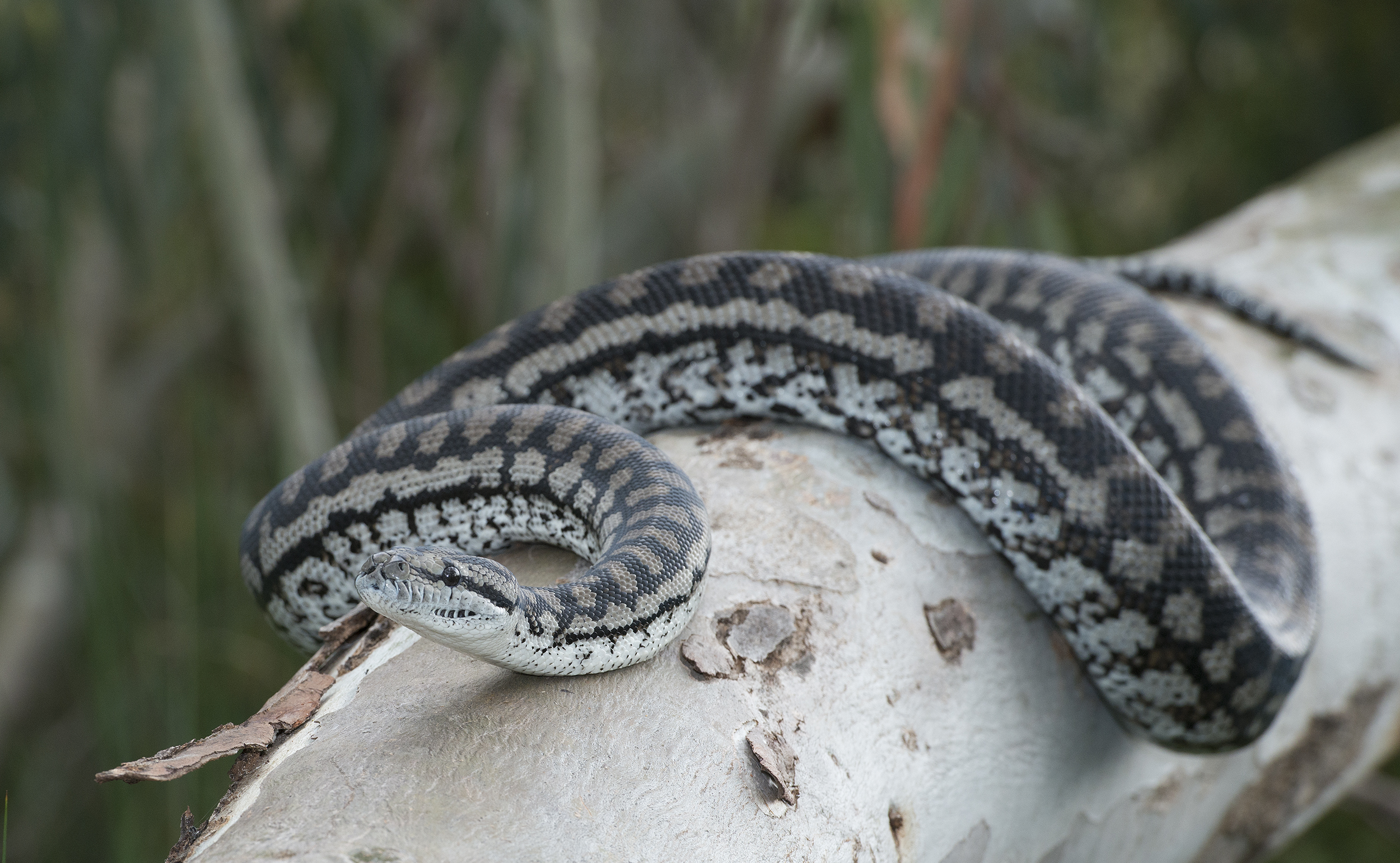The image features a gray and black snake with a complex pattern of brown squares and lighter tan lines along its top, while its underbody is predominantly white with black markings. The snake's scales are distinctly visible as it rests in a curled, serpentine position atop a white, rough-barked tree limb, likely a fallen branch. Its small, triangular head is lifted slightly, and it looks towards the center left edge of the photo, with its black eyes clearly visible. The background showcases a blurred forest, emphasizing the snake as the central focus of the photograph.